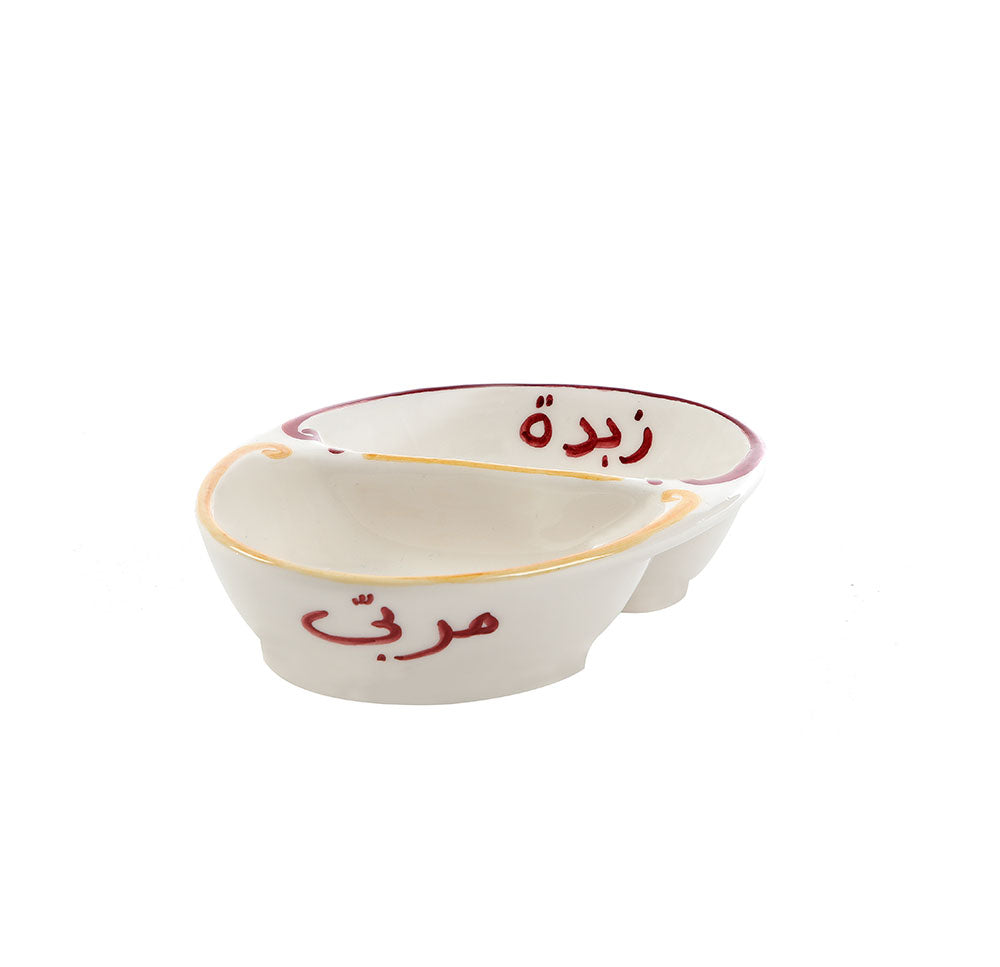The photograph showcases a white, ceramic dip bowl with two compartments, each shaped like a half-moon and divided by a central crease. The left compartment features a yellow line along its rim, while the right compartment has a pink or red line. Both compartments are adorned with red symbols in a foreign language, possibly Asian. Notably, the symbol inside the right compartment resembles the letter "O" with two dots above it, followed by a shape akin to the letter "J." The bowl rests against a plain white background, emphasizing its intricate design and dual functionality.